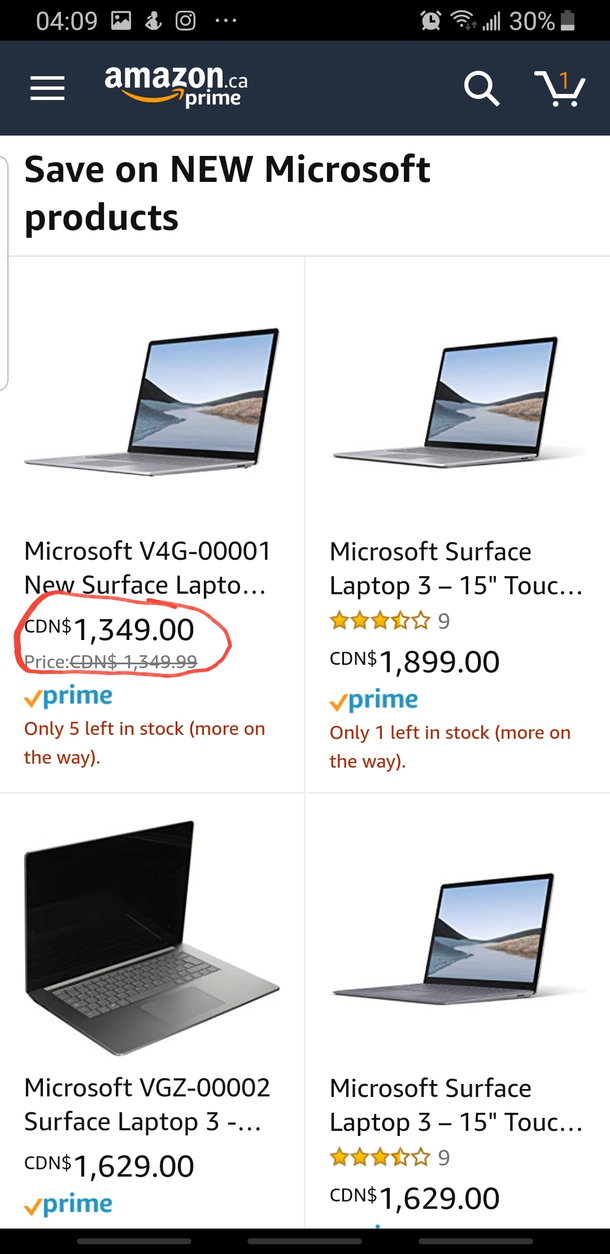The image depicts a webpage interface with various elements meticulously detailed. 

At the top of the image, there is a dark black banner displaying "4:09" in white text, indicating the current time. Adjacent to it, there is a gray outline icon featuring a black background with a small gray dot and a stylized representation of mountains. Beside it, there is an icon resembling a person running, followed by a camera icon with an ellipsis ("...") next to it. To the far right of the banner, several status indicators are visible: an alarm clock icon, a Wi-Fi signal icon, a cell phone signal icon, "30%" text indicating the battery level, and a battery icon. 

Below the top banner, the background lightens slightly, displaying three horizontally stacked white lines, which could symbolize a menu. Next to these lines, the text "amazon.ca prime" is prominently shown. To the right of this text, there are two icons: a magnifying glass symbolizing search functionality and a shopping cart with the number one inside it, possibly indicating one item in the cart.

Descending further, the background transitions to white with a bold header, "Save on new Microsoft products," where "NEW," "Microsoft," and "S&C" are all capitalized for emphasis. 

The following section is a panel displaying four distinct images of Microsoft products. The first image presents a laptop with the label "Microsoft V4G-00001 new Surface laptop" and a price of "CDN $1,349," encircled in red. The subsequent image's description reads "Microsoft Surface laptop 3 15 inch touch," but it's partially blacked out. The third product's text at the bottom of the image states "Microsoft VGC-00002 Surface laptop 3," with its position indicating it is at the top of the webpage. The last product's label, "Microsoft Surface laptop 3 - 15 inch touch," appears cut off, suggesting incomplete text or limited display space.

The webpage layout seems to provide a detailed and organized view of shopping options for various Microsoft Surface laptops, highlighting the essential features, labels, and prices, along with icons pertinent to the website's navigation and user interface.